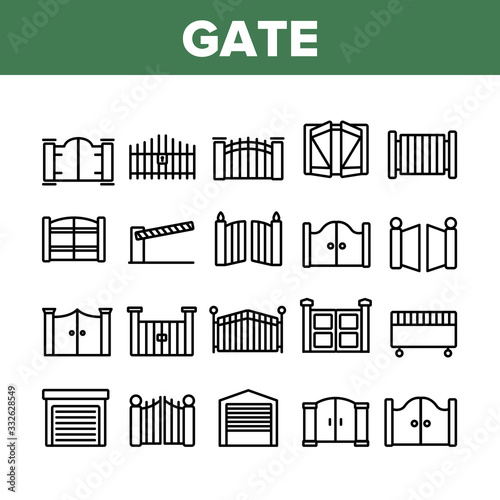The image features a collection of 24 detailed, black-and-white line drawings of various gate styles, arranged in four rows of five columns. These gates range from residential double-door designs to singular doors and include specialized gates like those typically seen at parking lots with raising and lowering arms. Above these illustrations is a narrow green horizontal bar with the word "Gate" prominently displayed in bold, white, angular block letters. The entire image is subtly watermarked with "Adobe Stock," which is particularly noticeable in the green area. In the lower-left corner of the image, the text “Adobe Stock #332-628549” is printed vertically.